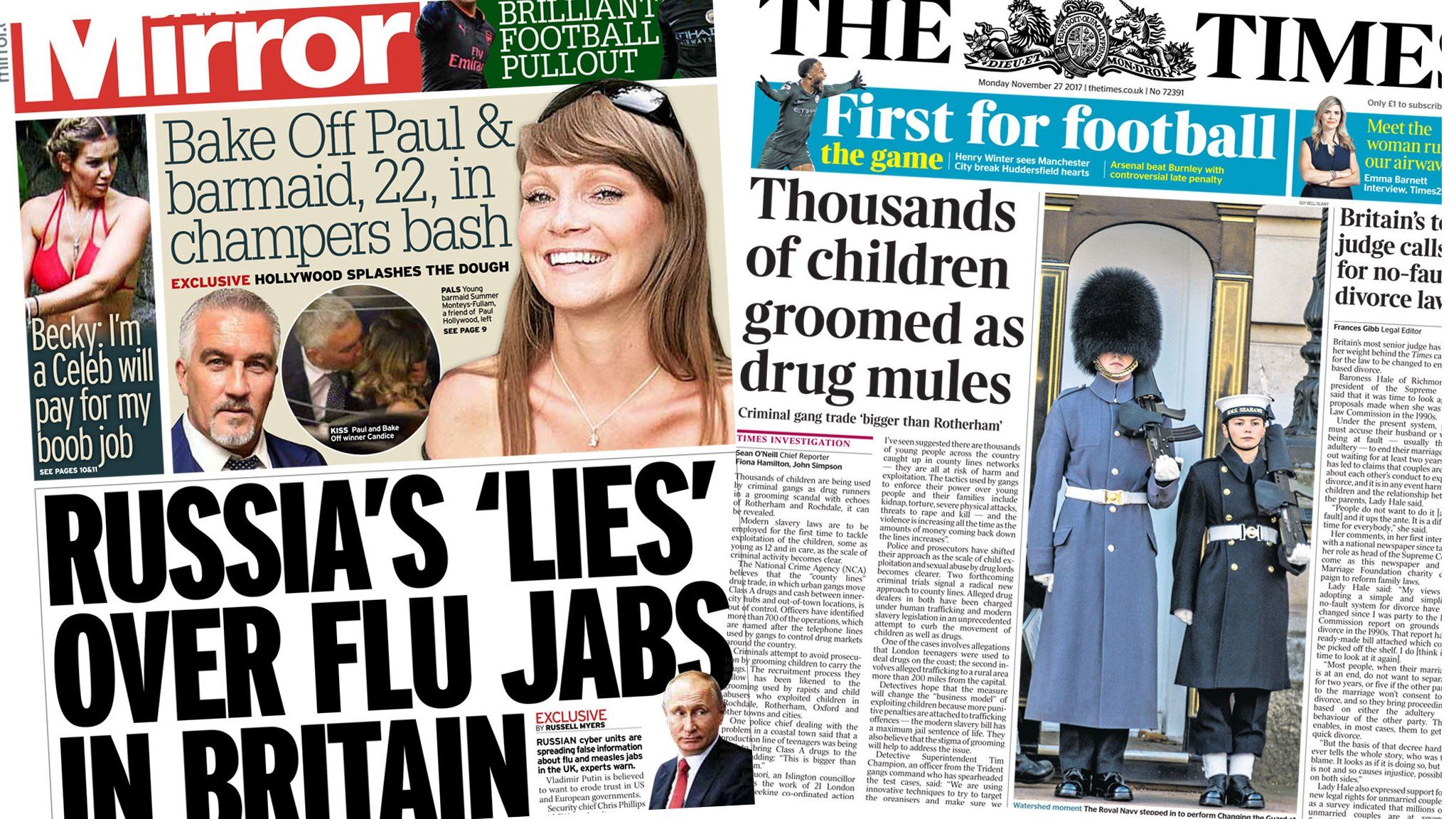The image features two magazine covers side by side.

**Left Magazine (Mirror):**
1. **Title and Headline**: The top section of the cover, in red, prominently displays the word **"Mirror"**.
2. **Feature Highlight**: A green section titled **"Brilliant Football Pullout"** is prominently displayed.
3. **Main Story**: The headline reads **"Bake-Off Paul and Barmaid, 22, in Champers Bash"**, with a subheadline stating **"Exclusive: Hollywood Splashes the Dough"**. An image shows a man and a woman kissing; the man is presumably Paul Hollywood. 
4. **Other Features**: 
    - An image of a woman in a bikini is present with an adjacent headline.
    - Below this, black text captures another headline: **"Russia's Lies Overflew Jabs in Britain,"** accompanying an image of Vladimir Putin.

**Right Magazine (Times):**
1. **Title and Headline**: The magazine title **"The Times"** is prominently displayed at the top.
2. **Feature Highlight**: It claims **"First for Football"** and **"The Game"**, featuring an image of a football (soccer) player.
3. **Main Story**: The headline reads **"Thousands of Children Groomed as Drug Mules,"**, with a subheadline stating **"Criminal Gang Trade Bigger than Rotherham"**. An article beginning is visible with **"Times Investigation"**, alongside an image of a man in a suit and a large, black fuzzy hat standing next to another person in similar attire, both holding guns.
4. **Additional Content**: There is an additional headline with an accompanying article and image below the main story.